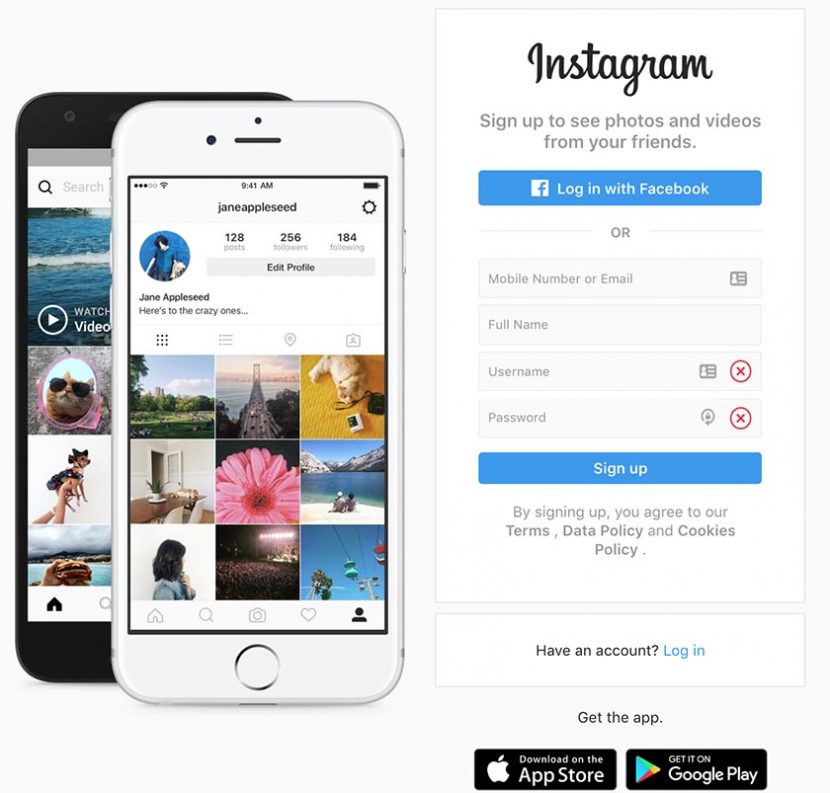This promotional image for the Instagram mobile app features a side-by-side comparison. On the left side, a white iPhone is prominently displayed with a black Android device slightly behind and to its left, showcasing the versatility of Instagram across different devices. Both phones display the Instagram app, featuring a grid of square thumbnails depicting a variety of photos, including flowers, landscapes, food, and pets, highlighting the diverse content shared on the platform.

The right side of the image presents a screenshot of the Instagram login and sign-up interface. The options for logging in include using Facebook via a blue button or by entering a mobile number or email, full name, username, and password for new accounts. Additionally, there's a direct login link at the bottom. The image concludes with a call to action, encouraging users to get the app through two prominent buttons for the App Store and Google Play. This detailed visualization emphasizes Instagram's user-friendly design and accessibility across multiple mobile platforms.